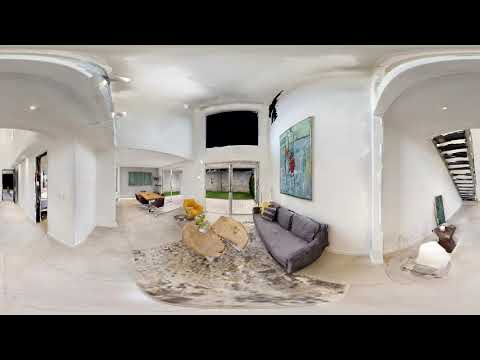The image depicts the interior of a modern apartment or house, captured in a somewhat distorted manner, as if taken with a 360-degree or surveillance camera, causing the lines to curve. The scene is letterboxed horizontally with black bars on the top and bottom, giving it a low-quality, blurry appearance. 

The walls and ceiling of the space are white, while the floor appears to be grayish concrete. Dominating the center of the image is a dark blue or purplish leather couch, stationed against one of the white walls. Above the couch hangs an abstract painting featuring a mix of blue, green, yellow, and red hues, its details unclear but vibrant.

To the right of the couch, there is a sliding glass door that opens to the outside. Hanging near the ceiling above this door is a large black rectangular object, most likely a flat-screen TV. 

In front of the couch, slightly to the center, sits a coffee table with an abstract design, and off in the distance ahead and to the left, a dining room table can be spotted along with another sliding glass doorway. The left side of the image also reveals a long hallway with multiple openings leading to other rooms.

To the right of the main seating area is a stairway leading upstairs, with modern abstract sculptures placed beneath it. Overhead, there are some lights illuminating the space. The entire scene ties together with a rug on the floor, which features a stony or abstract pattern, fitting well within the modern aesthetic of the room.